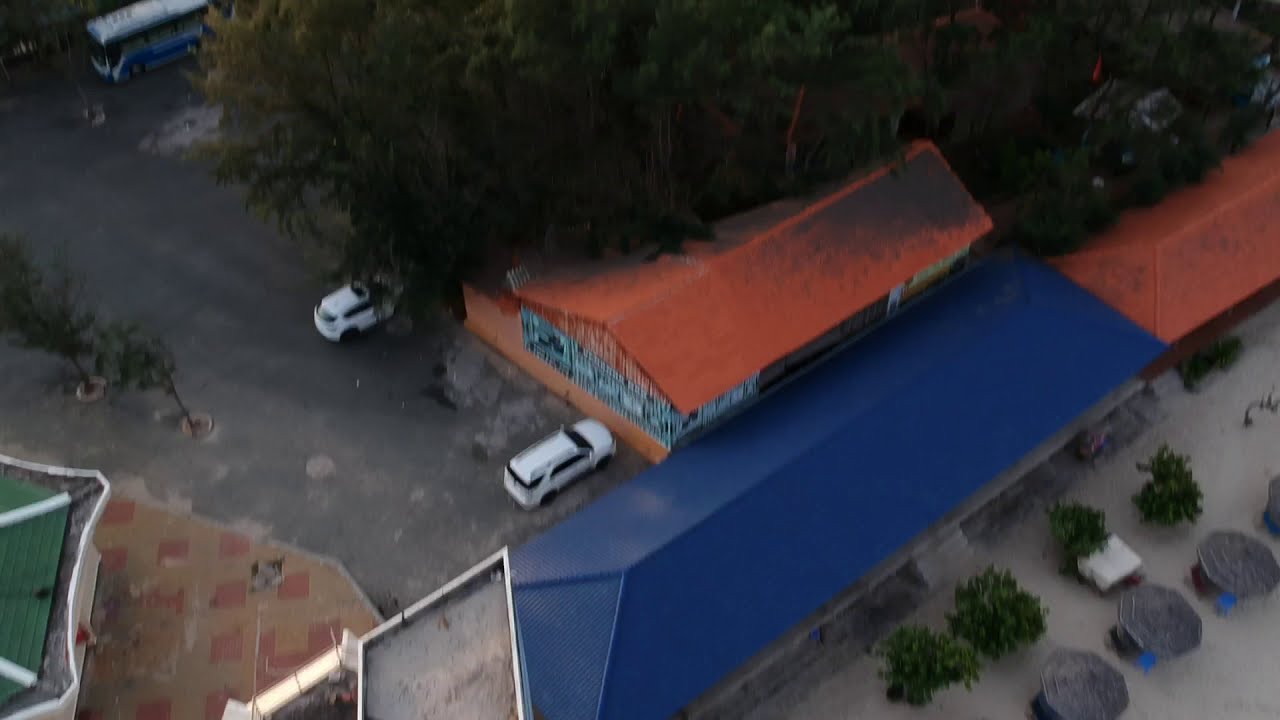This aerial photograph captures a vibrant scene dominated by houses with distinctively colored conical roofs. At the center of the image, there is a house with an orange roof. Adjacent to it, from the bottom to the top right of the picture, stretches a long house with a striking blue roof. Directly next to this blue-roofed house is another building with an orange roof. In front of the blue-roofed house, there's a small area featuring some plants and tables on a white-colored ground. There are two white cars parked near the orange-roofed houses, situated on a gray ground area. The scene is complemented by green trees scattered around the buildings. The arrangement of the buildings and the color palette give a lively contrast, with blue and orange roofs forming the central focus, interspersed with green foliage, the gray hue of the street, and white elements from the cars and certain areas on the ground. Notably, some of the buildings show signs of wear, with broken glass windows visible on one of the orange-roofed structures.